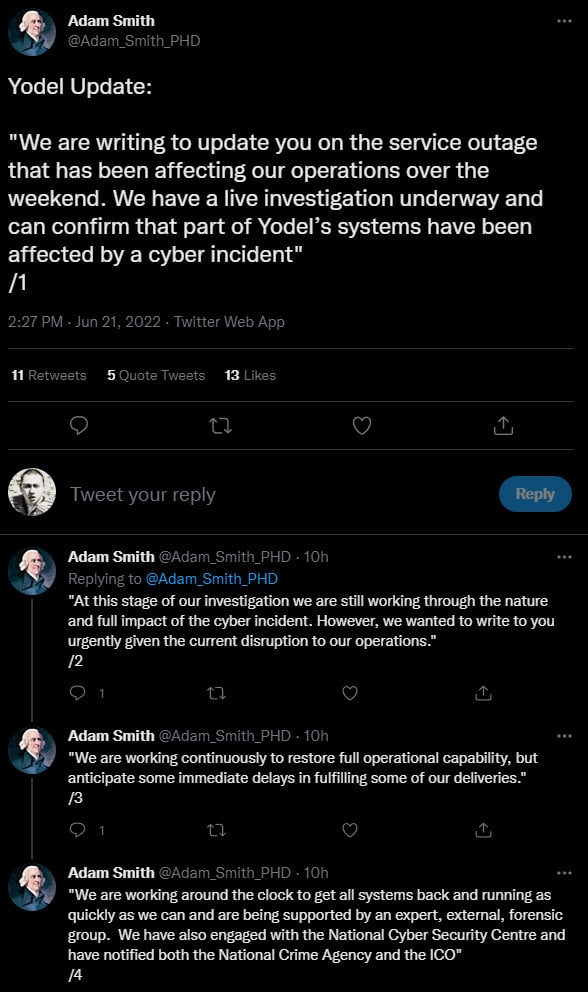**Caption:**

Screenshot of a Twitter update from Yodel regarding a significant service outage due to a cyber incident. The tweet, originally posted by Adam Smith on July 21, 2022, informs users about the ongoing investigation into the cyber attack that has disrupted their operations over the weekend. The tweet has garnered 11 retweets, 5 quotes, and 13 likes. Below the initial post, there are four subsequent updates providing more information: 

1. Confirmation of the cyber incident affecting Yodel's systems.
2. An update on the current stage of their investigation and efforts to understand the full scope and impact of the incident.
3. An assurance that efforts are being made continuously to restore full operational capability.
4. A reaffirmation of their commitment to getting all systems back up and running as soon as possible.